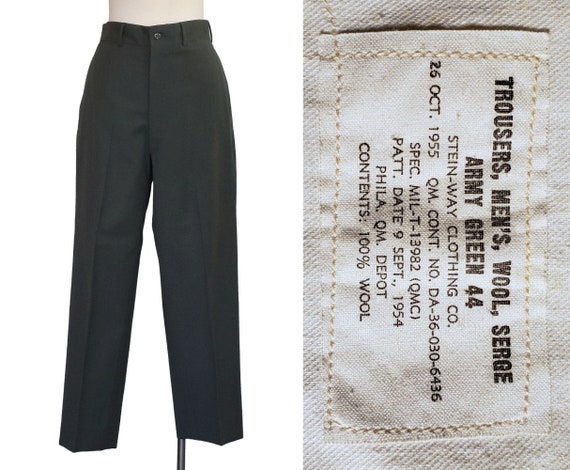The image displays a pair of black trousers fitted on a beige-topped mannequin, showcasing the front with belt loops, a black button, and a front crease, indicative of casual or possibly black jeans. The trousers are set against a white background. To the right, there is a detailed close-up of the trousers’ white linen label affixed inside, oriented sideways. The label reads: "Trousers, Men's, Wool, Serge," followed by "Army Green 44" centered beneath. Below this is "Steinway Clothing Company," the date "26 October 1955," and additional text including "QM count number DA360306436," "Spec Mill T13982," "Pat Day 9 September 1954," and "Fila QM Depot." The material content is noted as "100% wool."